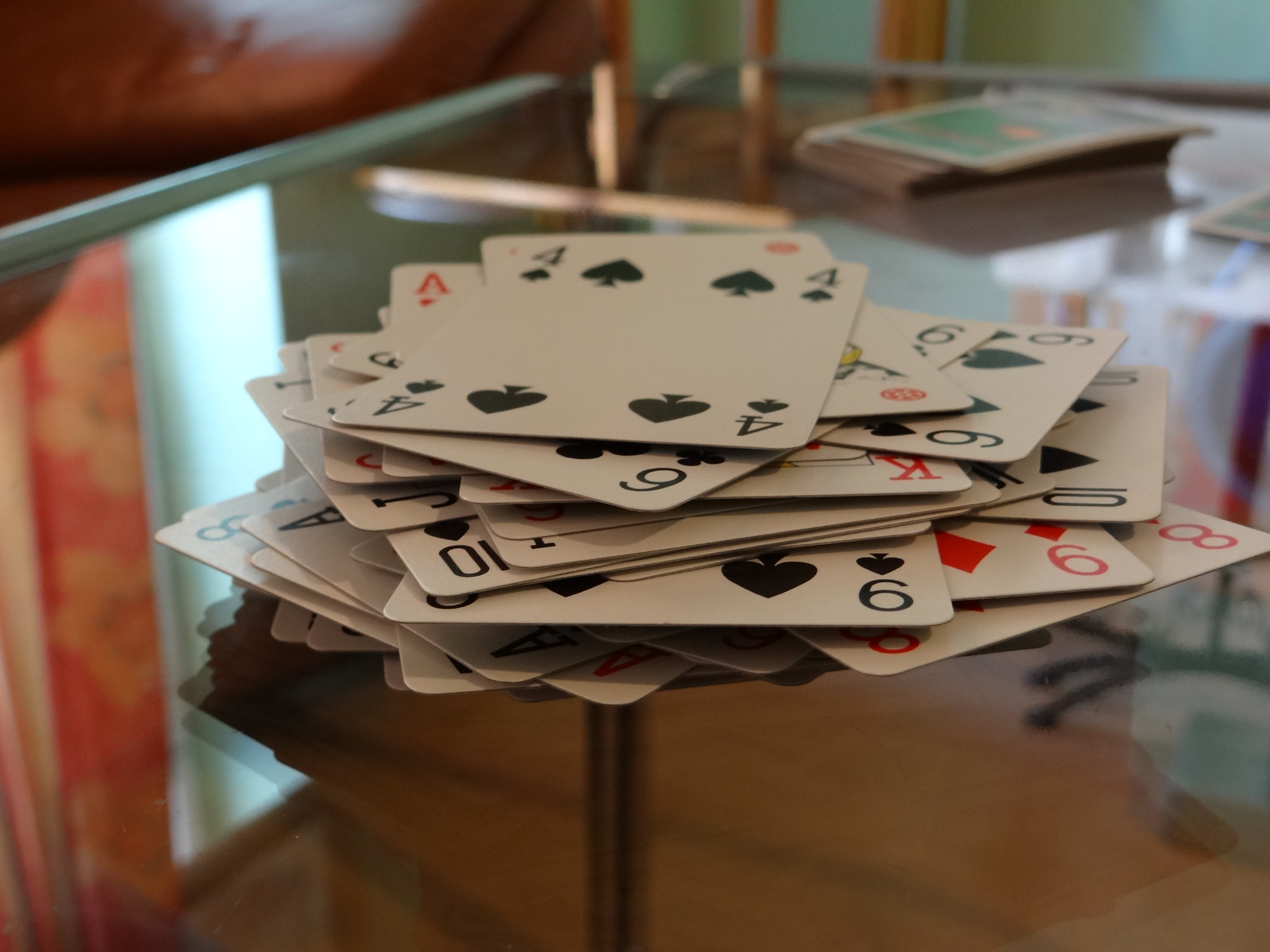This detailed photograph captures a clutter of playing cards resting atop a glass coffee table. Prominently visible in the foreground are a four of spades, a six of clubs, a six of spades, a ten of spades, and a nine of diamonds. Several other cards, including an eight and an assortment of eights and aces, are stacked closely together, making it difficult to discern their suits.

Surrounding the pile of playing cards, the glass table also hosts a few green cards with white borders. These are positioned towards the background, with their finer details obscured due to distance and angle.

In the backdrop, a reddish-brown piece of furniture adds a warm hue to the scene, while on the opposite side of the table, a black, wheeled stool partially enters the frame. 

Notably, the reflective surface of the glass table captures intriguing reflections. Adjacent to the reddish-brown furniture, the table mirrors the edges of the playing cards, and within this reflection, a vibrant item featuring a red background coupled with a floral pattern is subtly visible.